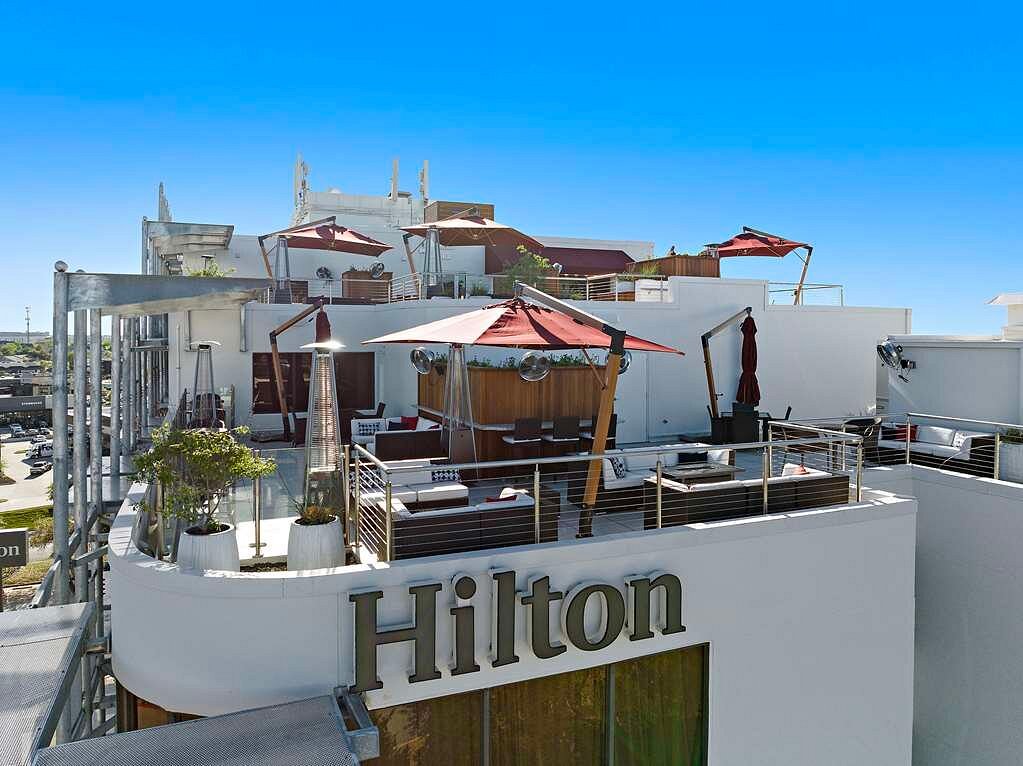This detailed rooftop view of a Hilton Hotel showcases an elevated outdoor leisure space featuring brown sofas adorned with white cushions, strategically arranged under elegant canopies and accompanied by outdoor heaters. The multi-leveled terraces are enclosed by railings and glass, ensuring safety while offering unobstructed views of the surrounding landscape. Notable elements include green potted plants adding a touch of nature, and a bar or cabana area for serving drinks. The rooftop area is reminiscent of penthouse suites, distinguished by orange and white umbrellas shading various seating arrangements. The iconic white building prominently displays the Hilton name, with a pristine blue sky, devoid of clouds, serving as the backdrop. The distant scene reveals the hotel grounds with patches of grass, pavement, and scattered cars, extending towards the horizon.